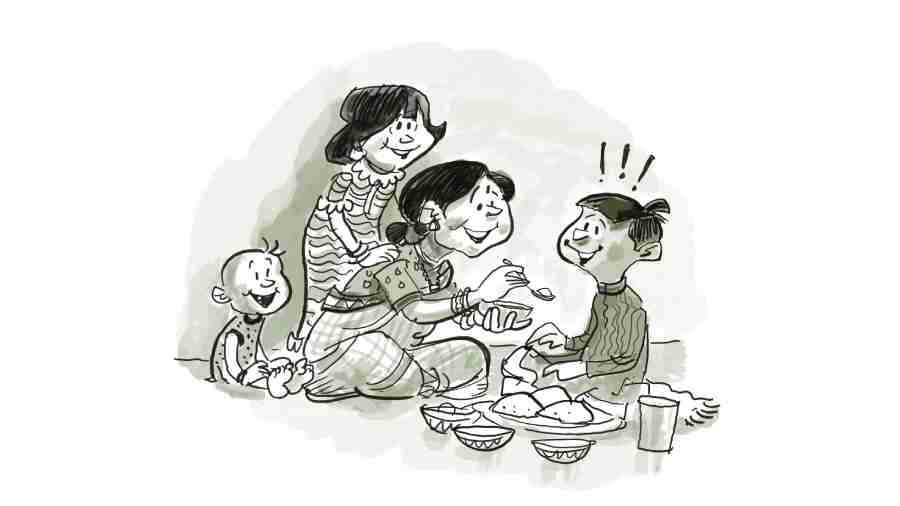The drawing depicts a warm family scene featuring a young mother seated cross-legged on the floor, engaging in a tender moment with her two children. Positioned in front of her is a little boy, eagerly awaiting his next bite as the mother, adorned in overalls with a shirt underneath and her black hair pulled back into a ponytail, holds a spoonful of food towards him. The child is visibly excited, as illustrated by three exclamation points above his head. Beside him on the floor lies a plate of food, surrounded by three bowls and a cup with a straw.

Nestled beside the young boy is a toddler with a few strands of hair drawn on his head, showcasing a single tooth in his cheerful smile. He watches intently, clearly anticipating his turn to be fed.

Behind the young mother, an older woman, presumably her mother, stands with a gentle, supportive smile. She has her hands reassuringly placed on her daughter's shoulders and is dressed in a striped dress adorned with ruffles at both the collar and the short sleeves. Her short black hair frames her face, which radiates warmth and affection as she witnesses the nurturing interaction. The drawing brilliantly captures the essence of generational love and familial support.